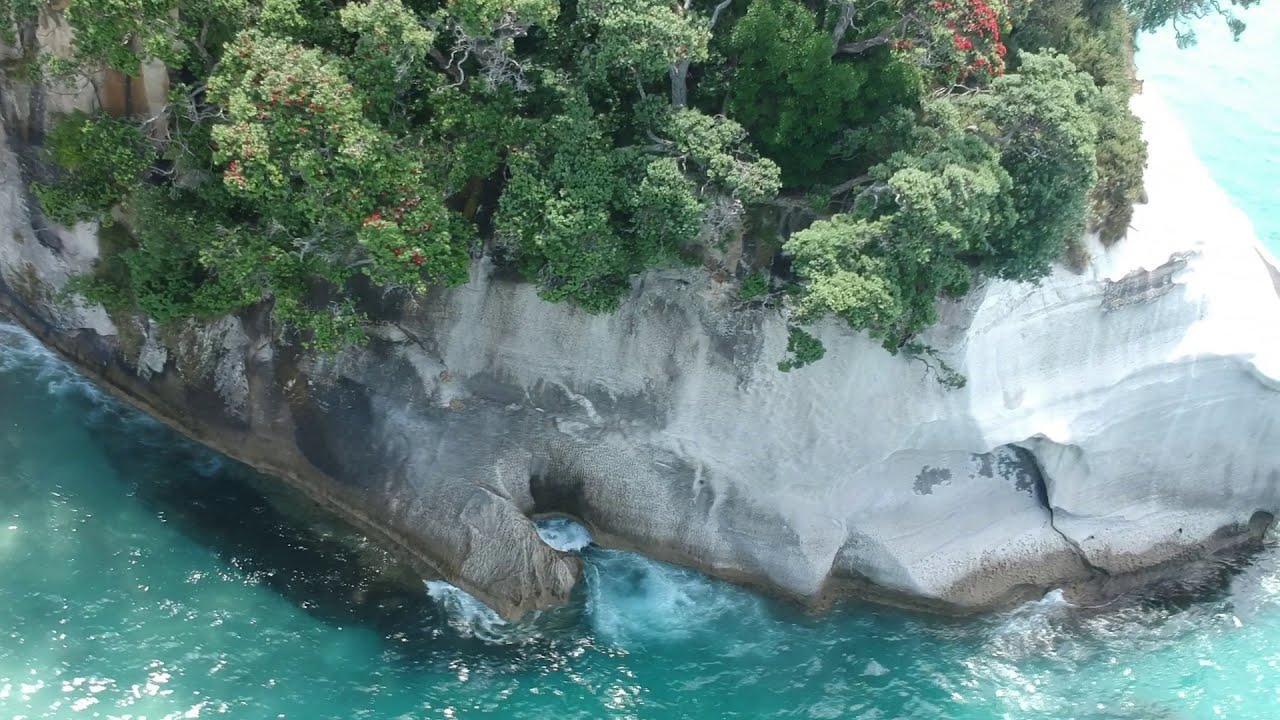The image depicts a stunning, rocky coastline adorned with lush, green trees and vibrant flowers. A massive, gray and black rock formation, about 20 feet tall, rises dramatically from the clear, turquoise ocean. This rocky cliff, featuring shades of gray and brown, seems to be bathed in sunlight on the upper right-hand corner, creating a contrast with the darker, shadier lower left. A splash of pink flowers adds a splash of color to the midsection, while red flowers mingle with the dense, dark green foliage atop the cliff. The ocean, with its mesmerizing blue-green hues and gentle waves, laps against the base of the cliff, and in the distance, the horizon merges seamlessly with the light blue, almost white sky.